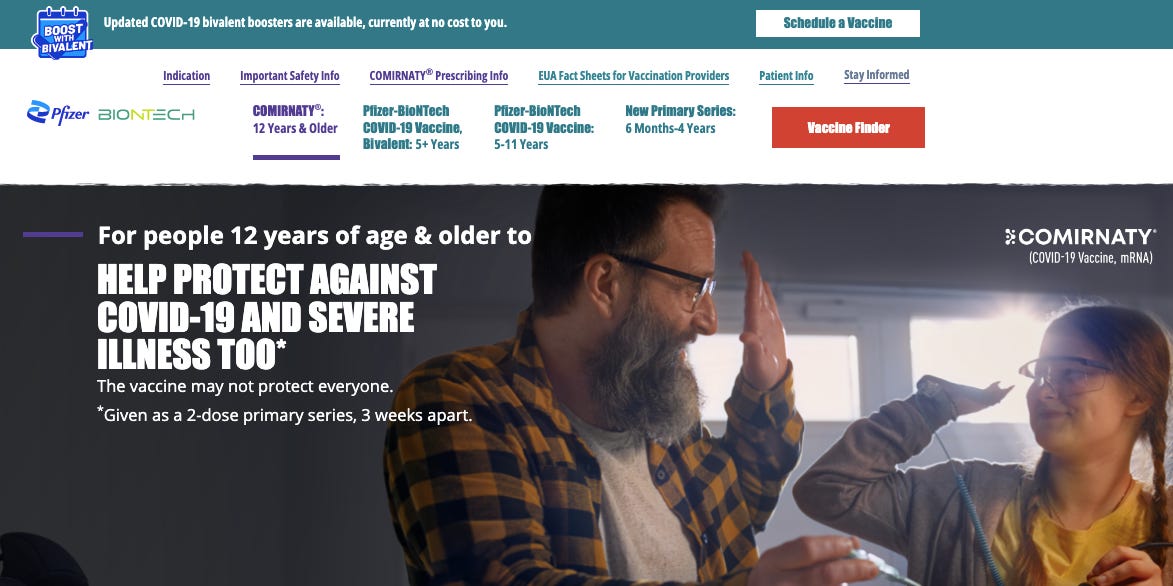In the top left corner of the image, there is a blue sticky note with white text that reads "Post with Pimvalent." To the right of this note, there is an update message stating, "COVID-19 Pimvalent posters are available currently at no cost to you." The date and text are in white over a slightly blue background. Adjacent to the update, there is a white button with dark blue text that says "Schedule a Vaccine."

Below this section is the main body of the page, featuring a white background. At the top are several tabs, "Indication," "Important Safety Info," and "Community Prescribing Info," all written in purple. In dark blue text are "EUA Fact Sheet for Vaccination Providers," "Patient Info," and "Stay Informed." Below these tabs, on the right side, there is a red button with white text that reads "Vaccine Finder." To the left of this button, in dark blue text, it reads "New Primary Series: 6 months - 4 years." Further to the left, it states "Pfizer BioNTech COVID-19 Vaccine: 5 to 11 years." Next to it, the text announces "Pfizer BioNTech COVID-19 Vaccine Pimvalent: 5+ years." Further left, it mentions "Community: 12 years and older."

To the far left, there are the company names "Pfizer" in blue and "BioNTech" in green and yellow. At the bottom of the image, a photograph shows a male (right side) and a female (left side) holding hands. The accompanying text on the left side reads, "For people 12 years of age and older to help protect against COVID-19 and severe illness too. The vaccine may not protect everyone. Given as a two-dose primary series, three weeks apart," written in white. Above this, on the right, it states, "Community COVID-19 Vaccine mRNA."